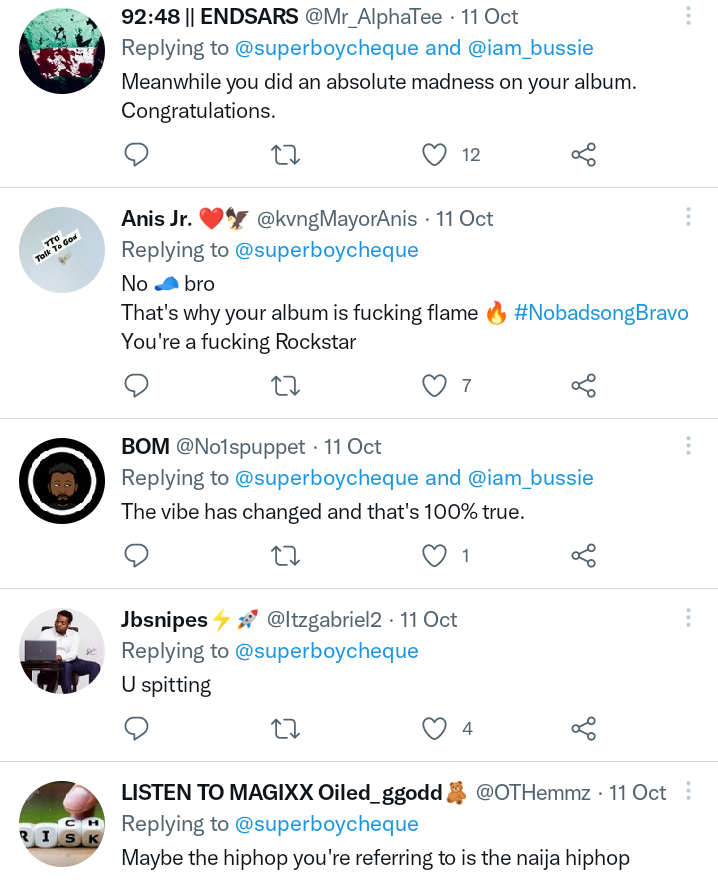Below is a detailed and cleaned-up caption for the given image:

---

The image shows a series of posts and replies on X (formerly known as Twitter), centered around user interactions with Superboycheck. 

1. **Nsars** (@Nsars) replied to Superboycheck and I_am_bussy, praising Superboycheck's new album: "You did an absolute madness on your album. Congratulations!"
2. **Anis Jr.** (@AnisJr) also responded to Superboycheck, extolling the album's quality with enthusiasm: "That's why your album is 🔥. You're a fucking rock star!"
3. **Bomb** (@Bomb) joined the conversation, replying to Superboycheck and I_am_bussy, echoing the sentiments: "The vibe has changed and that's 100% true."
4. **JB Snipes** (@JBSnipes) kept it concise in their reply to Superboycheck: "You spit."
5. Finally, **Listen to Magics** (@oiled_G_God) commented, suggesting a geographical specificity: "Maybe the hip hop you're referring to is Naija hip hop."

The cohesive dialogue highlights the overwhelmingly positive reception of Superboycheck's new album among his followers.